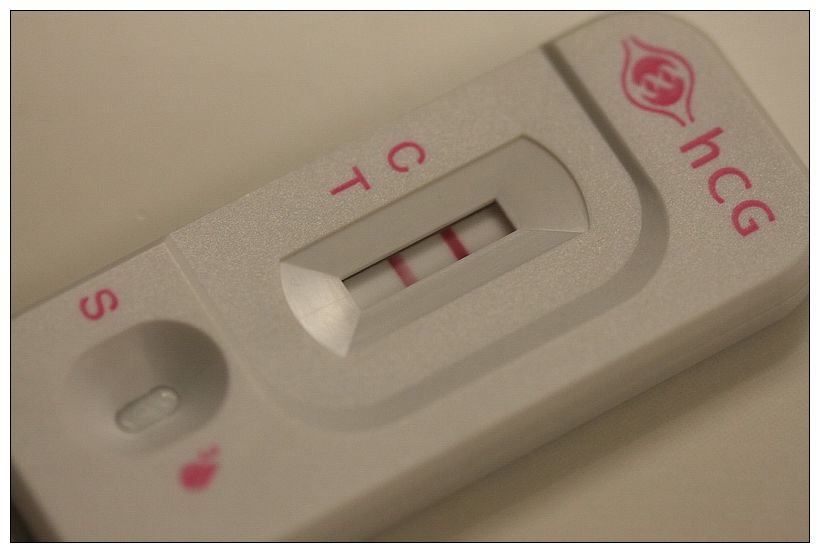This image features an extreme close-up of a white testing strip placed on a white surface. The testing strip is elongated and narrow. At the top of the strip, there is a bulbous shape colored in pink, which has a design in its center. Adjacent to this pink bulb-like symbol are the letters "hCG" with a lowercase 'h' and uppercase 'C' and 'G'. 

Moving down the strip, there is a small window containing two horizontal bars labeled 'C' and 'T'. The 'C' bar is a darker pink, indicating the control line, while the 'T' bar is a lighter pink, suggesting a positive result for whatever this test is designed to detect. 

Further down, there is an 'S' marked along the side of the strip, next to another small opening likely meant for inserting the sample. On the opposite side of the 'S', there is a pink marking that appears fuzzy and out of focus, making it indistinguishable.